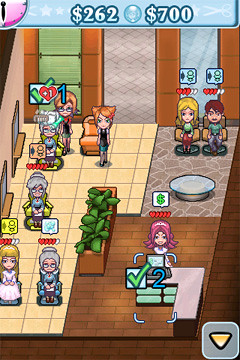This screenshot captures an interior scene from a video game, depicting avatars positioned throughout a diverse environment within a building. The room is divided into sections with varied textures: some areas have tiled floors, others feature stone, and additional portions are wooden. In the background, a brown hue dominates, providing a warm, cohesive backdrop. Each avatar is seated in distinct chairs scattered across the room, highlighting the room's different zones. Above each character's head float several hearts, indicative of their current health or vitality level, along with icons that display various unique symbols representing different statuses or abilities. The interface also includes a blue banner at the top of the screen, displaying the figures "$262" and "$700," which likely denote in-game currency or scores. Additionally, a directional arrow icon is present in the bottom right corner, suggesting a navigational option or pointer within the game.